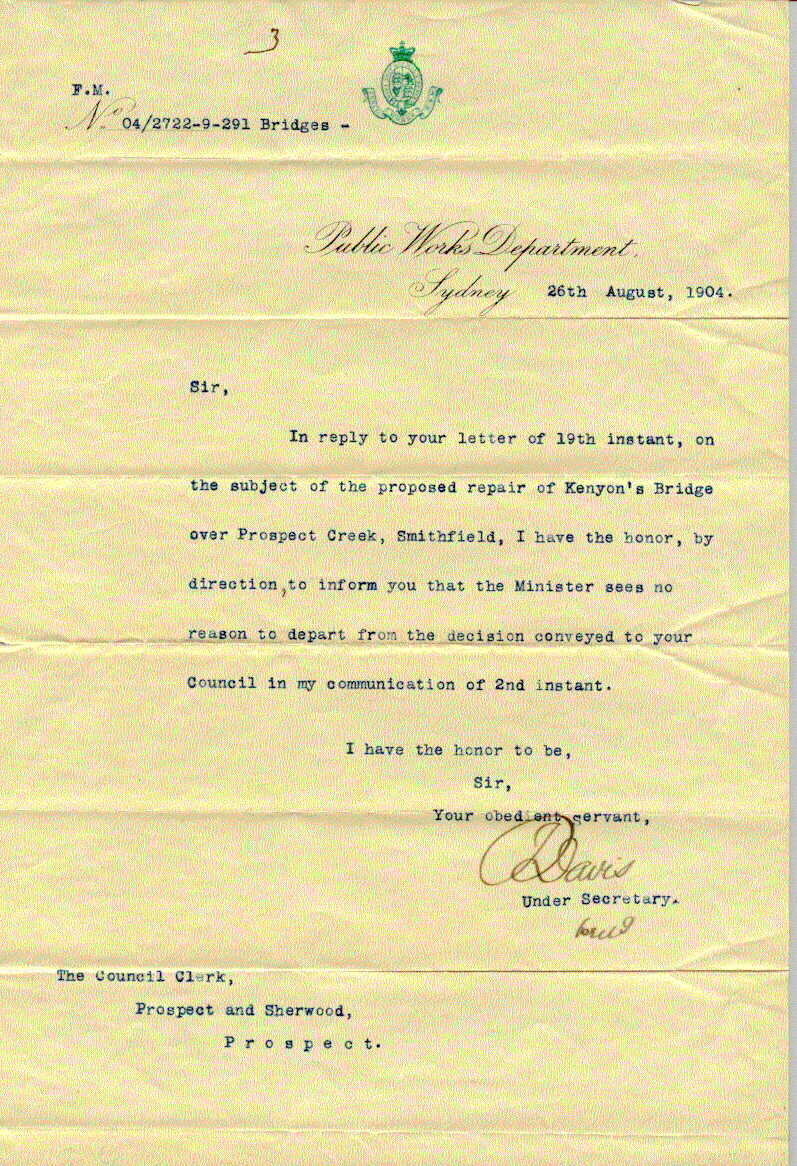This photograph captures a piece of light yellow stationery paper featuring a green logo at the top, which consists of a circle with a ribbon beneath and a crown atop it. In the upper left-hand corner, the letters "FM" are printed, followed by "N" in cursive script. The inscription "04-2722-9-291 Bridges" appears below. The document originates from the Public Works Department in Sydney, dated 26 August 1904. The main content of the letter is typewritten in black ink and addressed to concerns about the proposed repairs of Kenyon's Bridge over Prospect Creek in Smithfield. The message states that the minister sees no reason to change a prior decision conveyed to the council. The letter is formally closed with the phrase "I have the honor to be, sir, your obedient servant," and signed in cursive, though the signature is indecipherable. Additionally, in the lower left-hand corner, there is a mention of the Council Clerk of Prospect and Sherwood, Prospect. The letter is over 120 years old.